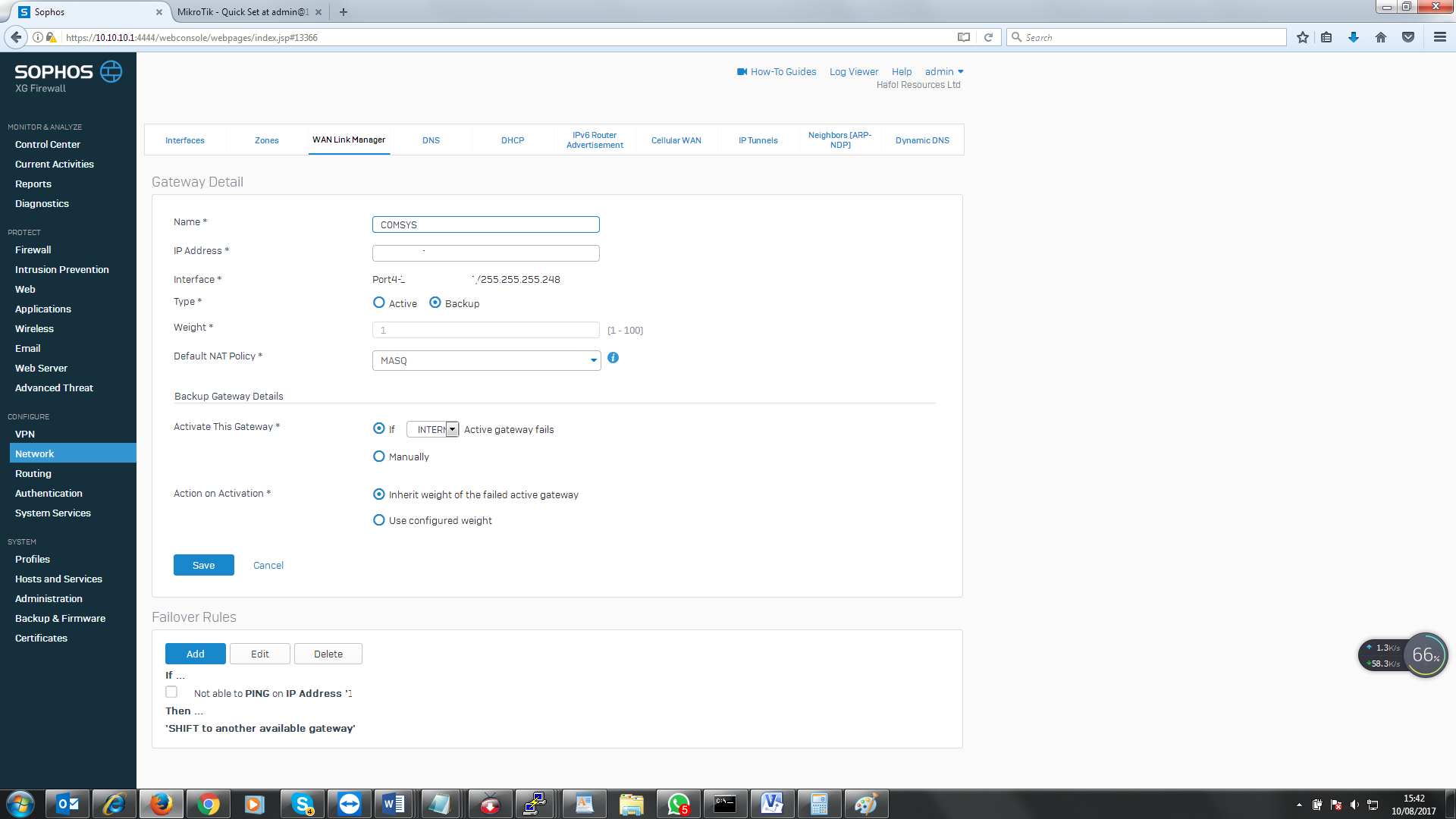A detailed, cleaned-up caption for this image:

“This screenshot captures a user navigating the Sophos website on a web browser, which is not identified as Chrome. The browser features a URL field, a large search bar to the right, a star icon for bookmarking, a 'Download Home' button, and a hamburger menu. The interface includes a dark vertical sidebar on the left, displaying several menu options. Although the labels are unclear, they seem to reference the 'Control Center,' 'Current Activities,' and sections like 'Firewall,' 'Email,' 'Web Server,' and 'VPN.' The selected and highlighted option, presumed to be 'Network,' is in blue. On the right side of the screen, there is a detailed section with numerous submenus, possibly including a 'Link Manager' and details regarding a 'Gateway' configuration. This area contains fields for entering a name, which appears to be 'combyS,' along with IP address, interface type, and various checkboxes, drop-down menus, and buttons for settings. At the bottom, there are blue 'Save' and white 'Cancel' buttons, as well as options to 'Add,' 'Edit,' and 'Delete' follower rules. The Windows taskbar is visible at the bottom, indicating the PC is running a Windows operating system.”